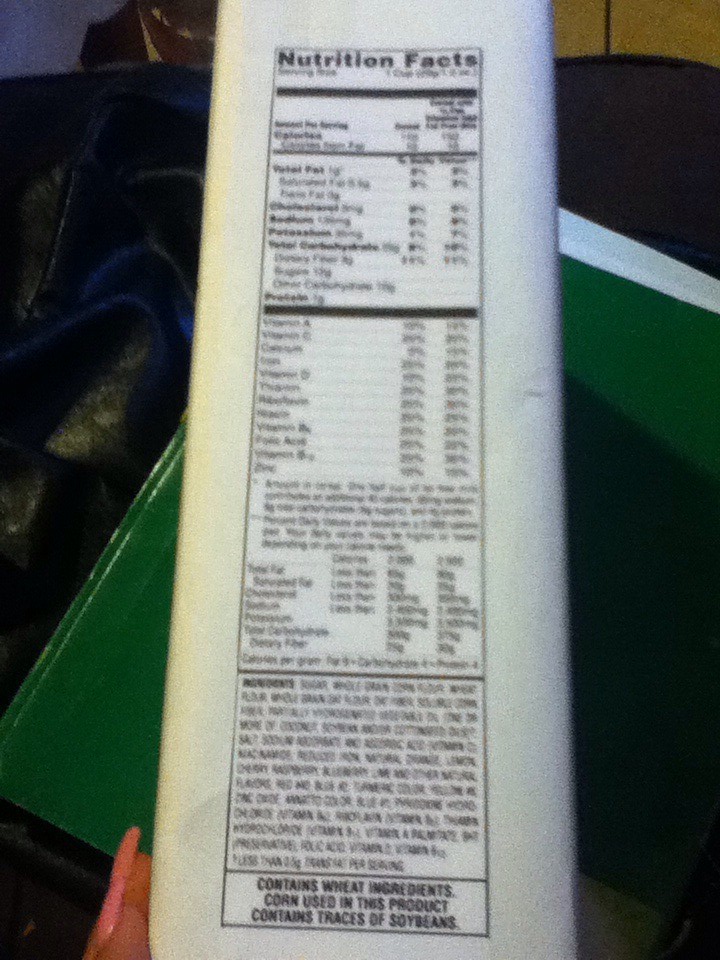In a realistically captured vertical photograph, an indoor room serves as the backdrop, adorned with disparate objects. The upper left side features a dark gray wall, transitioning to light brown wood paneling on the upper right. The central background is a mix of darker areas alongside a green surface, possibly a folder tilted to the right with a white sliver of paper protruding from it. Towards the bottom left, two fingers with long, pink-colored fingernails are visible. These fingers are holding a tall, slender white object centrally positioned in the image. This object appears to be either a plastic bottle or a food box, characterized by an extensive label. The label contains a large black-bordered rectangle with "Nutrition Facts" at the top, followed by several horizontal lines segmenting out various nutritional details. Though blurry, it appears to list macronutrients, vitamins, and ingredients, with notable mentions of wheat ingredients and traces of soybeans.